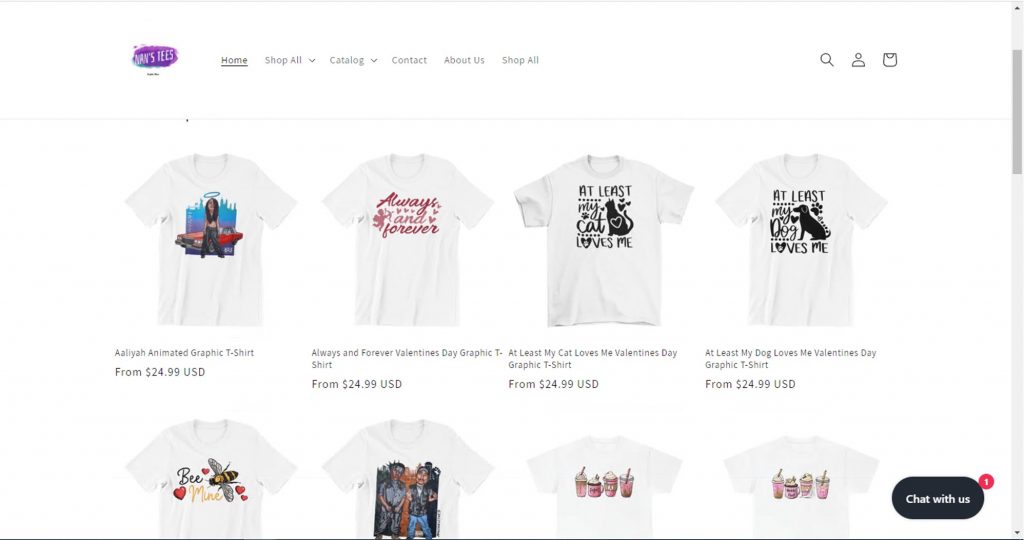This image showcases the homepage of a shopping website named "NAN TEES." The logo is prominently displayed in purple and white, with the letters "NAN" in white against a purple background. The website's navigation menu includes several options: Home, Shop All (with a drop-down menu), Catalog (also with a drop-down menu), Contact, About Us, and Shop All. Additionally, there is a search icon represented by a magnifying glass, a login option, and a shopping cart icon to view added items.

The homepage features a grid of eight T-shirt images, each priced starting from $24.99 USD. The displayed T-shirts include:
1. An Aaliyah animated graphic T-shirt.
2. An "Always and Forever" Valentine's Day graphic T-shirt.
3. An "At least my cat loves me" Valentine's Day T-shirt.
4. An "At least my dog loves me" Valentine's Day T-shirt.
5. A "Be Mine" T-shirt featuring an illustration of a bee.
6. A T-shirt with images of rap artists Biggie Smalls and Tupac Shakur.
7. Two identical T-shirts depicting four different beverages, likely coffee or frappes, without any accompanying text.

At the bottom of the screen, there is an option to chat with customer support. A notification icon is also visible, indicating that there is one unread message or alert.